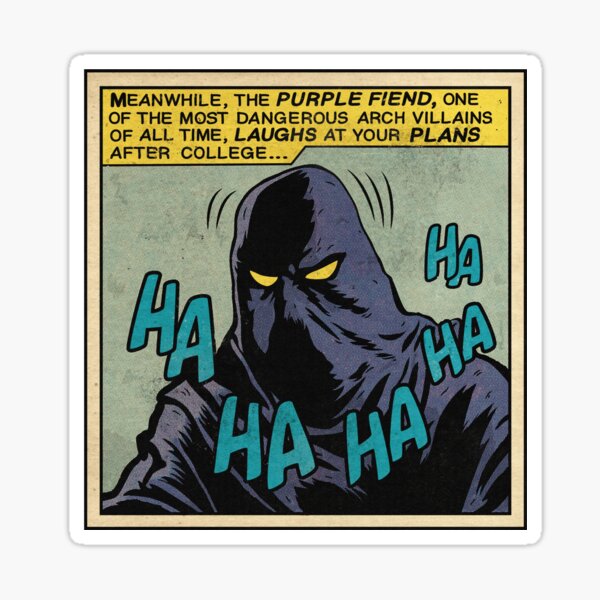The comic book panel features a dark-hooded figure known as the Purple Fiend, one of the most dangerous arch-villains of all time, laughing menacingly at your plans after college. The Purple Fiend, centered in the image, has bright yellow eyes that stand out against his ominous, dark attire. Around his head, five large "Ha, ha, ha, ha, ha" in purple letters emphasize his evil laughter. The entire panel is square, bordered first by a white frame and then a tan inner border. At the top of the panel, a yellow text box with black, all-capital letters reads, "Meanwhile, the Purple Fiend, one of the most dangerous arch-villains of all time, laughs at your plans after college..." Key phrases such as "Purple Fiend," "laughs," and "plans" are bolded and italicized for emphasis. The overall style is reminiscent of a classic comic book section.